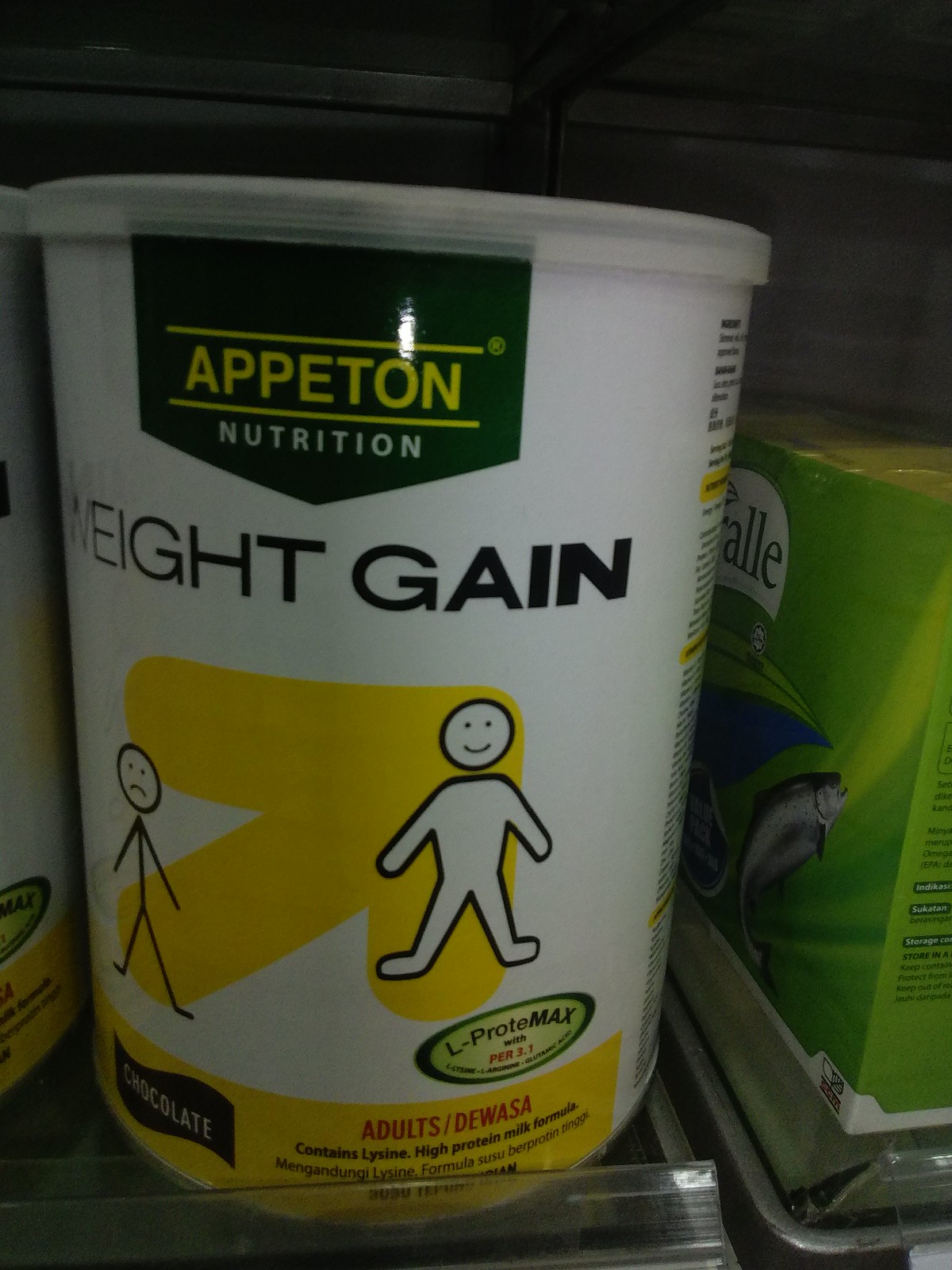The image depicts a white cylindrical canister of Apeton Nutrition Weight Gain, prominently displayed on a store shelf. The canister, which appears to be made of plastic, features a clear lid and distinctive branding. The label on the container is detailed: "Apeton" is written in yellow on a green background, framed by white lines above and below, followed by "Nutrition" in white. Beneath this, "Weight Gain" is printed in bold black letters. A large yellow arrow points to the right, illustrating a transformation from a lean stick figure with a frown to a bulkier figure with a smile, symbolizing weight gain. Further down, the label includes "Chocolate" and "Adults," along with a description indicating it contains lysine, high protein, and milk formula. Flanking the canister are other products, including a green cardboard box with a fish graphic on it, adding context to its placement in a retail environment.